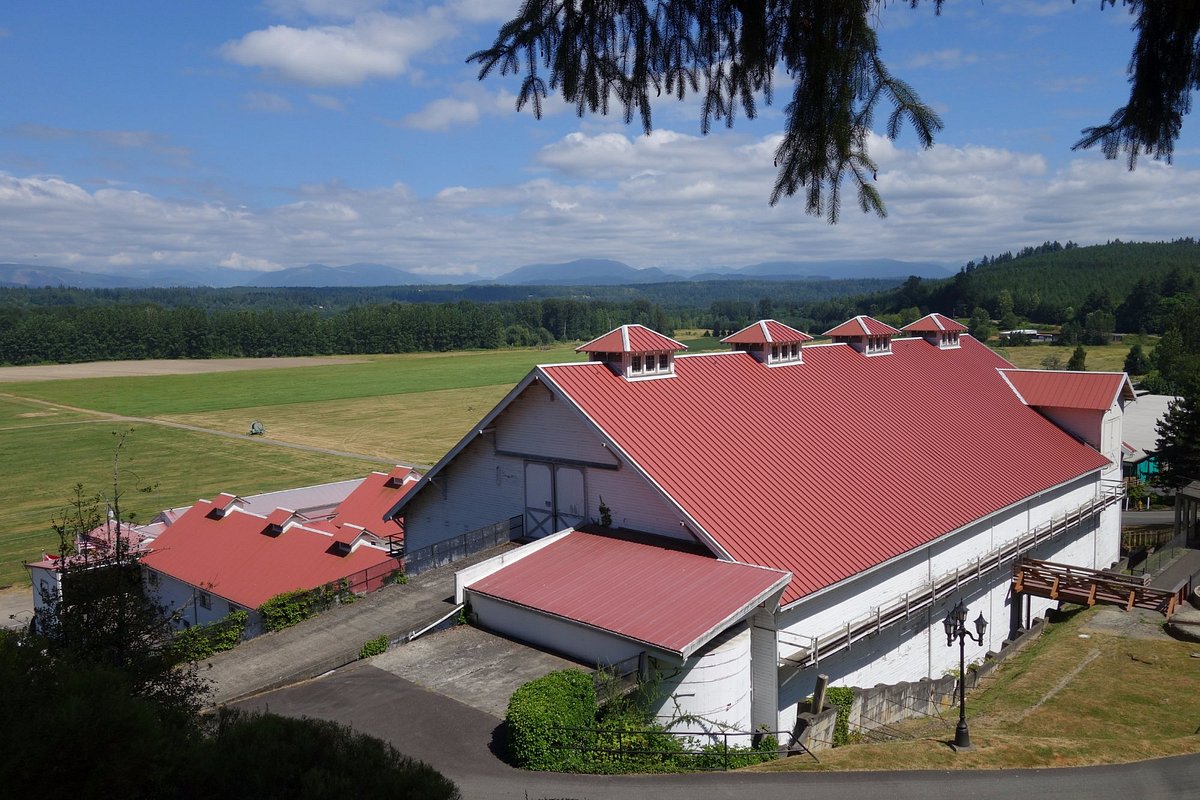A large, weathered barn dominates the center of a rural, farm-like setting. The barn features striking white walls and an arched, steeply angled metal roof that is a vibrant orange hue. Atop the barn are four small, ventilated sections, each with four holes, arching centers, and orange roofs similar to the main structure. An angular extension with an amber-colored roof and a white rim juts out from the bottom left side of the barn.

To the left, additional similar buildings can be seen, mimicking the primary barn’s shape and colors, each adorned with birdhouse-like structures on top, featuring the same orange roofs with white lines. The surrounding area is characterized by open green fields and clusters of dark green trees. A road weaves from the front of the barn outwards, hinting at connectivity with the wider rural landscape.

In the distance, rolling hills and scattered mountains create a picturesque backdrop under a bright blue sky dotted with white clouds, suggesting a sunny day in either spring or summer. No animals or humans are immediately visible, though there's a faint image of what might be someone on a tractor far in the background. The overall scene exudes a serene and timeless agricultural ambiance.